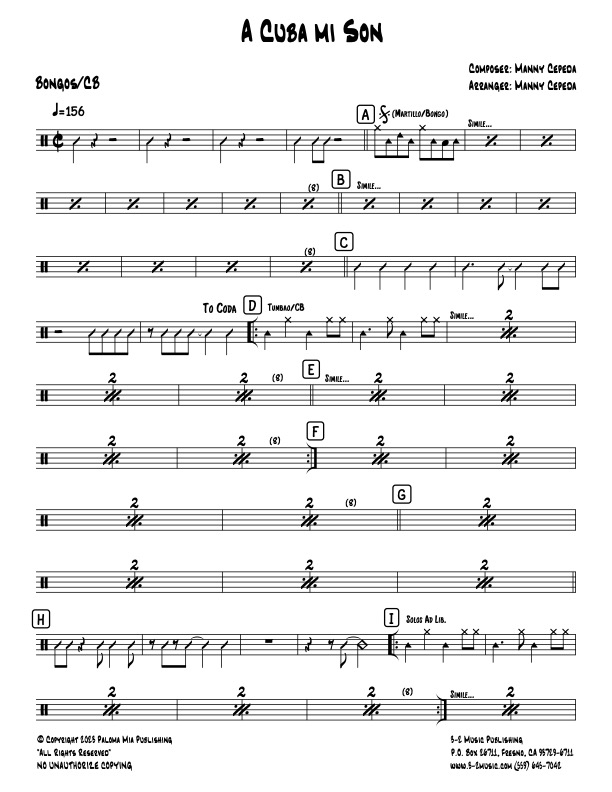The black and white image features a piece of sheet music titled "Akusa Mi Son." The composer and arranger, Nani Sepeda, are noted at the top right. The score includes approximately 10 lines of musical notation, each labeled with letters from A to I. The tempo is marked as 156, and the time signature indicates a combination of quarter notes and eighth notes, suggesting a rhythmic piece, possibly for bongos. At the bottom left, the copyright information is dated 2023 and attributed to Holomania Publishing.